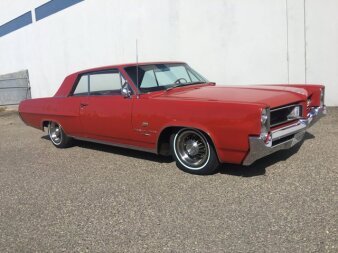The photograph captures an early 1960s style red car, characterized by its large "boat" body and distinctive features. This antique vehicle, viewed from the right-hand side with its front grillwork facing the observer and rear end angled towards the upper left, has white wall tires and silver hubcaps. It sits on a tan gravel or brownish concrete surface outdoors, in front of a white building accentuated by a blue stripe at the top. The building, which resembles a warehouse, has high-placed steel gray window-like strips on the top left corner. The image, possibly an old square photograph, lacks the sharpness typical of digital photos, adding to its vintage feel.